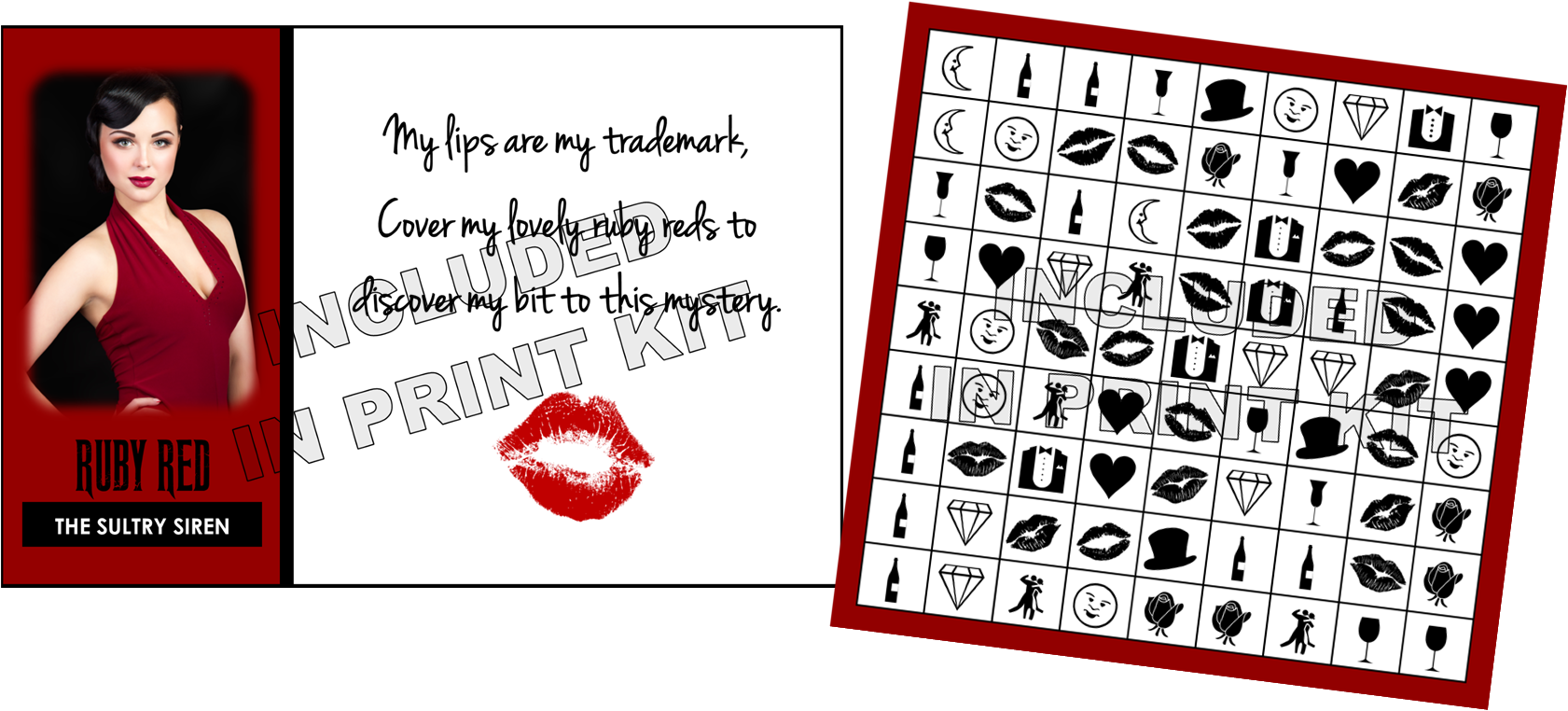The image showcases two pieces of paper placed side by side. On the left is an evocative image of a white woman with short black hair, clad in a red halter top dress, embodying a vintage noir aesthetic. She has striking red lips that add to her sultry look. Beneath her image, the text in black reads, "Ruby Red, the Sultry Siren," against a red background. Adjacent to this, in the white part of the card, it says in black script text, "My lips are my trademark. Cover my lovely Ruby Reds to discover my bit to this mystery," and a lipstick imprint sits just below the text. Both the image and text have a watermark reading, "Included in print kit."

To the right of this, there is another paper resembling a bingo card with a nine-by-nine grid of various black and white icons. These icons include lipstick lips in various angles (some closed, some open), crescent moons, wine bottles, wine glasses, hearts, smiley faces, diamonds, tuxedos, top hats, roses, and a couple dancing. This card also has a red border and bears the same watermark stating, "Included in print kit." The arrangement of these elements suggests an engaging, possibly interactive, component likely tied to a mystery game.